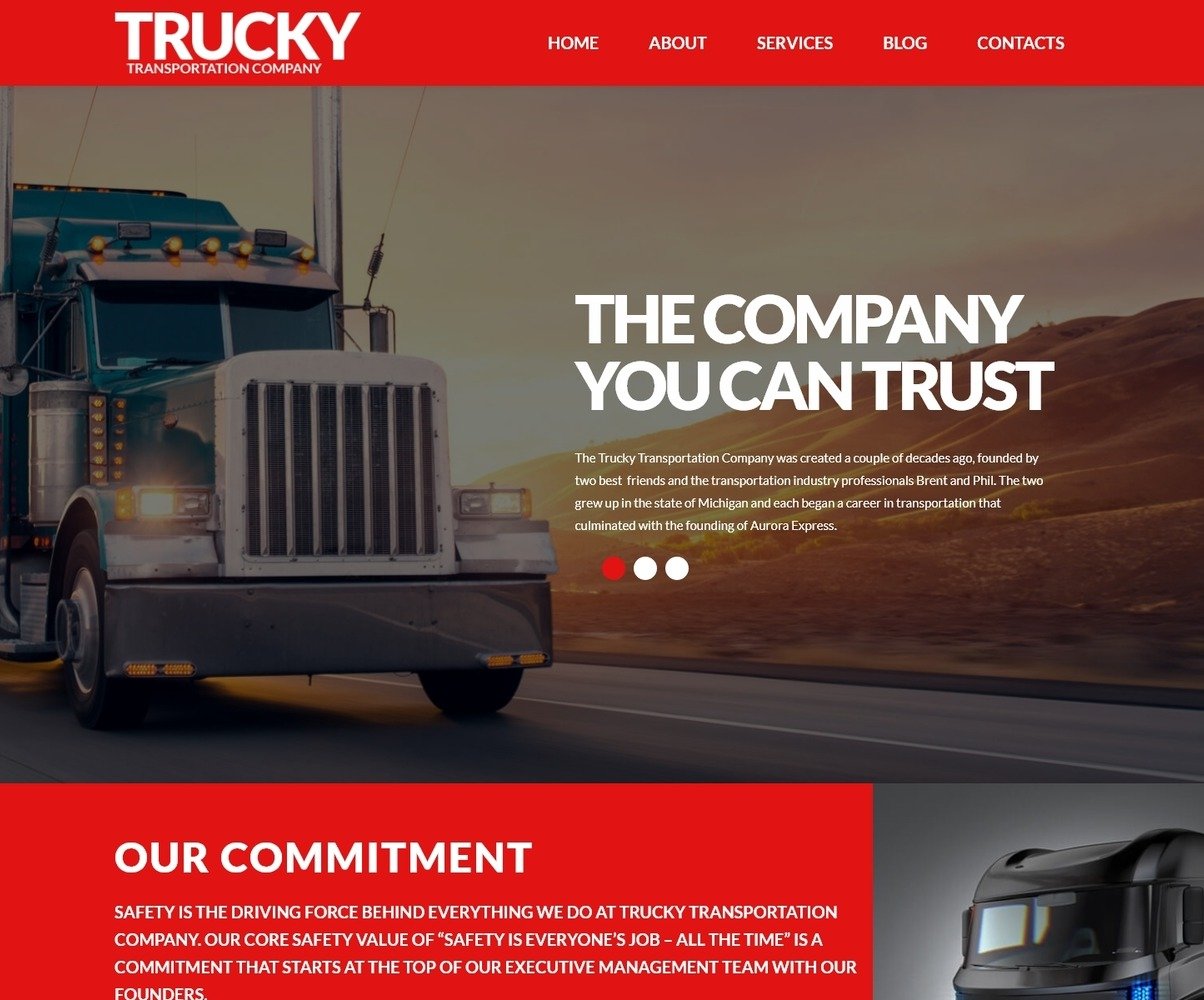This image showcases the homepage of Truckey, a transportation company. Featured prominently is a striking red header bar, where the company’s name, "TRUCKEY," is displayed in large, bold white capital letters. Directly beneath, in smaller uppercase white letters, is the descriptor "TRANSPORTATION COMPANY." 

To the right within this vibrant red header, the navigation menu items—Home, About, Service, Blog, and Contacts—are displayed in a clean white text. 

Beneath the header, the central image of the homepage captures a powerful red truck, prominently positioned with its two front wheels visible on the left side. Adjacent to the truck, a compelling tagline "THE COMPANY YOU CAN TRUST" is written in large, bold white text.

Below this central imagery, a rectangular text box spans approximately three-quarters of the page width. This box, also in white text, bears the heading "OUR COMMITMENT" in capital letters, followed by a detailed description of Truckey's dedication to its clients, set in smaller uppercase font.

The overall layout is visually engaging, highlighting both the robustness of Truckey’s brand and the commitment they bring to their transportation services.